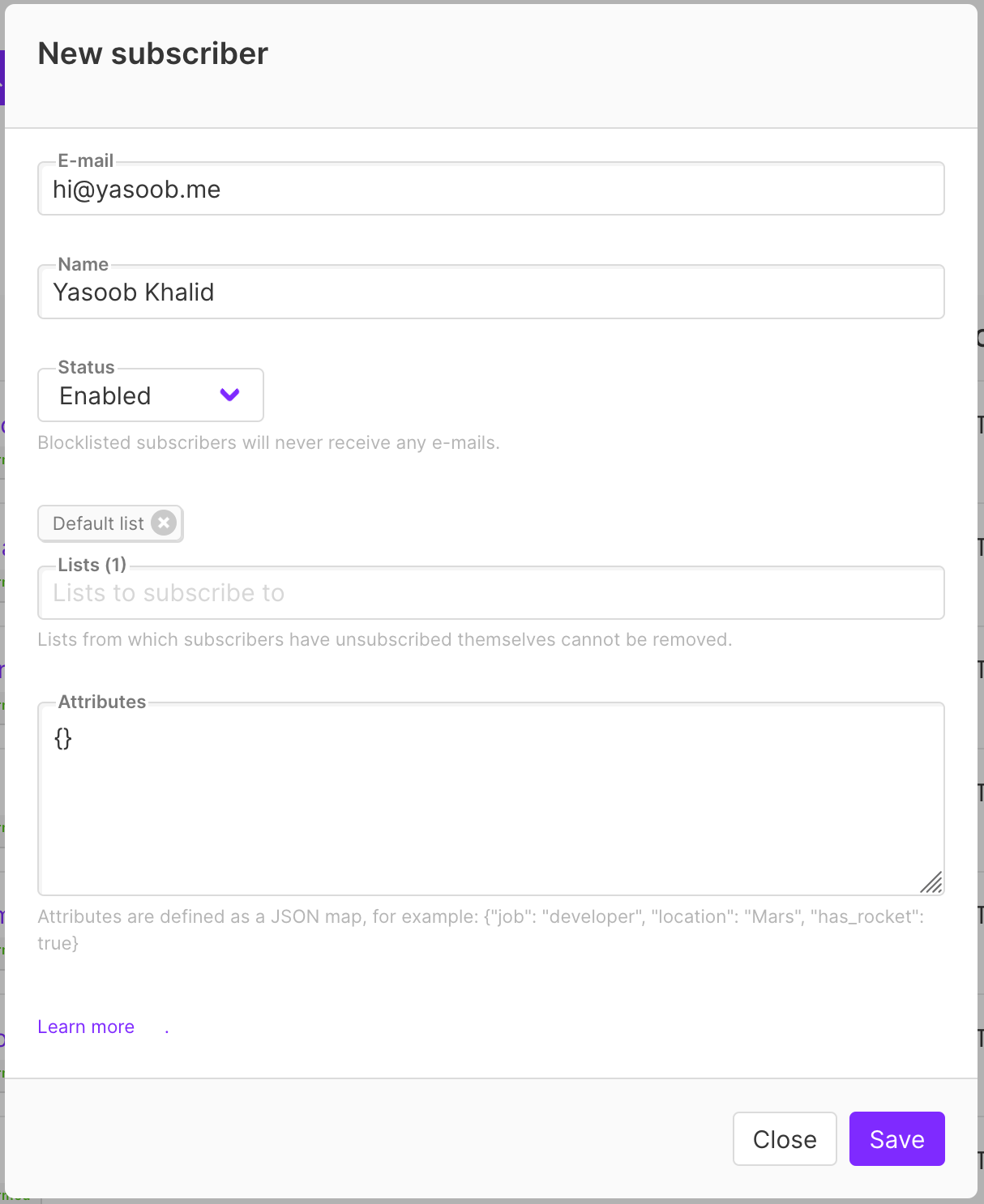A pop-up window appears on a webpage, prompting users to subscribe by filling out their details. The form includes fields for an email address, a name, and a subscriber status. Currently, it shows an email "hi@yassoub.me" and a name "Yassoub Khalid," with the subscription status as "enabled." The pop-up seems oriented towards subscribing to various lists, suggesting that it could be a newsreader service or app. Users can choose which news feeds to subscribe to from a "Default List." Additionally, there is a section labeled "Attributes," which allows users to specify their interests via a JSON map format. For example, "job: developer, location: Mars, has rocket: true," which could help tailor the news feed to display more relevant content based on the user's interests. The overall design and information are quite basic, focusing primarily on subscription management and personalization through user-defined attributes.